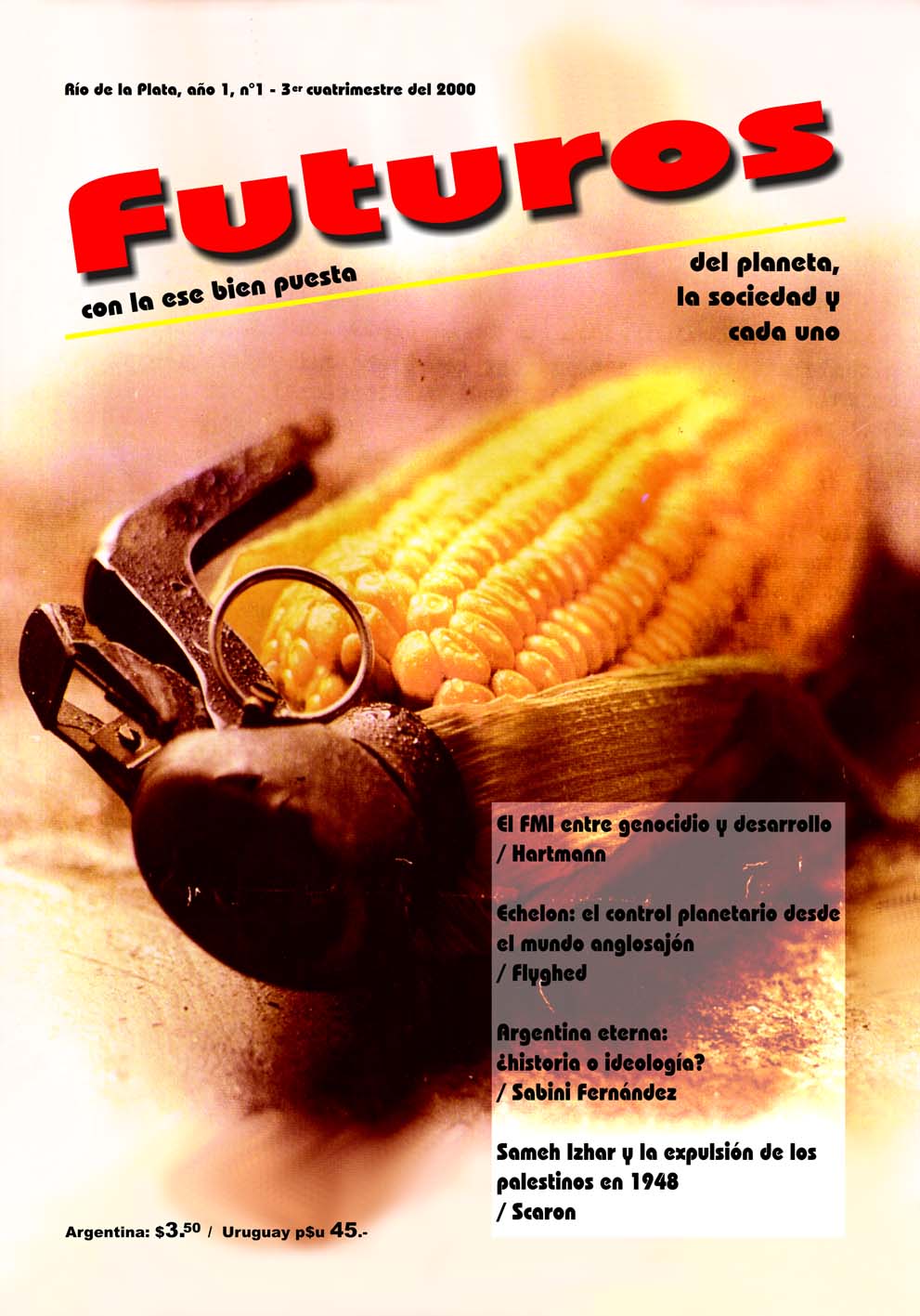The cover of a magazine or book prominently displays an ear of corn, partially husked and horizontally laid on either a table or natural dirt ground. Filtered to give an antiquated appearance, the image focuses on a peculiar detail: a metal item, possibly a bottle opener or the head of a hand grenade, embedded into the cob, suggesting an explosive or emerging effect. Dominating the cover is the slanted title "FUTUROS" in large red letters, underlined by a yellow line, with black drop shadows enhancing the font. Below, in contrasting black and brighter text, it reads "CON LA ESE BIEN PUESTA, DEL PLANETA LA SOCIEDAD Y CON EL UNO," hinting at themes beyond culinary content, potentially touching on serious issues like genocide. Additional text includes "Rio de Plata Anyo 1-3" at the very top left corner, pricing information "Argentina $3.50 / Uruguay $4.50" at the bottom, and smaller print "Argentina $3.50 / Uruguay P $45." The right-hand side features a large column of text, presumably continuing the discourse suggested by the subtitles.